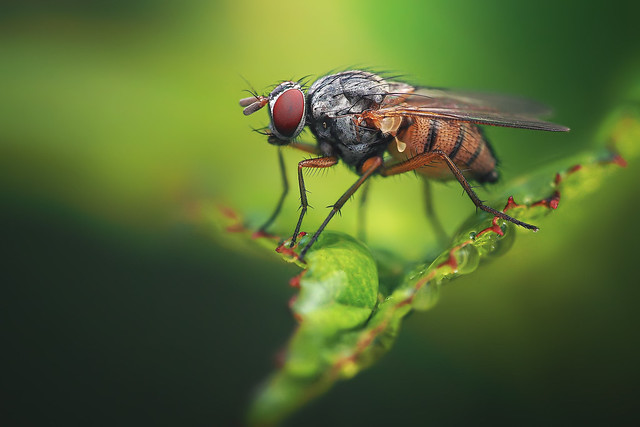This image is a professional, close-up photograph of a housefly standing on a green leaf with tiny red tips along its perimeter. The background is blurred in various shades of green, allowing the focus to remain on the intricate details of the insect and a portion of the leaf. The housefly, with its six legs, showcases distinct physical features: dark red, rust-colored large eyes; two short antennas or sensors protruding above its eyes; and delicate wings. Detailed examination reveals its orange lower body adorned with three black stripes stretching from back to belly, and the thorax, possibly featuring black spikes. The photograph captures the housefly's intricate anatomy and the textured surface of the leaf with remarkable clarity.